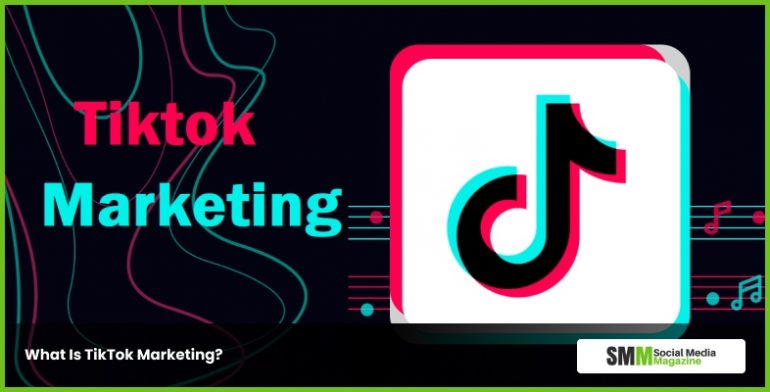This image is an advertisement or thumbnail for a video about TikTok marketing. It features a sleek, thin green border surrounding a primarily black background that incorporates dynamic patterns and lines in the signature TikTok colors: cyan, black, and red. Center stage, the text "TikTok" appears prominently in red, while "Marketing" is displayed in a striking blue font. 

Adjacent to this text, a large TikTok logo stands out against a white background. Underneath the logo, there's a semi-transparent banner that reads "What is TikTok Marketing?" in clean, white lettering. 

Towards the right side of the image, there's a small button or window marked "SMM Social Media Magazine." Here, "SM" is in black, the other "M" is in green, with the phrase "social media" written in small black font underneath, and "magazine" in green font below that. This landscape-oriented image is horizontally aligned, being much wider than it is tall.